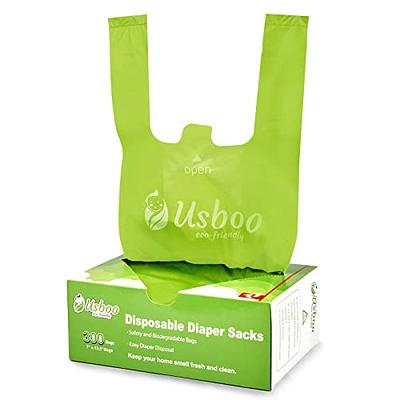The image features a box of USBOO Disposable Diaper Sacks against a blank white background. This green and white rectangular cardboard box is prominently displayed in the center of the image, with detailed text and branding. The box, designed for easy access, has a triangular opening at the top from which a single disposable diaper sack is visibly protruding. This sack is made of light yellowish-green plastic, similar to a grocery bag, and features two handles for convenient use. The sack displays the brand name "USBOO" and a small logo of a swaddled baby in white lettering. Additionally, the box is labeled with "Disposable Diaper Sacks USBOO 300 count," alongside phrases such as "safety in biodegradable bags," "easy diaper disposal," and "keep your home smelling fresh and clean." The side of the box, primarily green with some white, contains more text, some of which is not fully readable in the image.